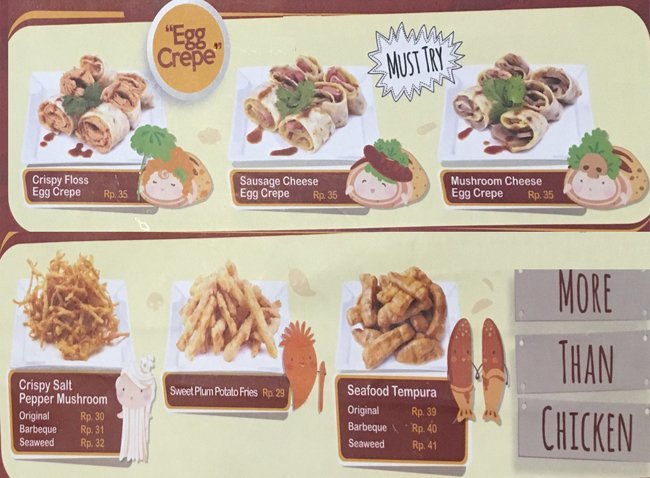The image depicts a photograph of a restaurant's menu board, taken from a slightly off-angle perspective. Dominated by a thematic yellow circle at the top that mimics an egg, the board advertises various egg crepe dishes. Inside the circle, "Egg Crepe" is prominently displayed alongside a small star icon containing the words "Must Try."

The menu features six distinct dishes, each paired with a corresponding photograph and a whimsical cartoon character resembling the dish. The offerings include:

1. **Crispy Floss Egg Crepe** (RP35) – A visual depiction of the crispy floss egg crepe.
2. **Sausage Cheese Egg Crepe**
3. **Mushroom Cheese Egg Crepe**
4. **Crispy Salt Pepper Mushroom**
5. **Sweet Plum Potato Fries**
6. **Seafood Tempura** – Available in original, barbecue, and seaweed flavors, accompanied by illustrations of fish-like characters.

The layout showcases three dishes across the top half and three across the bottom half of the board. In the lower right corner, gray rectangles feature the words "More Than Chicken," hinting at the nutritional value or perhaps the diverse offerings beyond just chicken. There is no indication of the location, but the variety and presentation suggest an inclusive, possibly international menu.